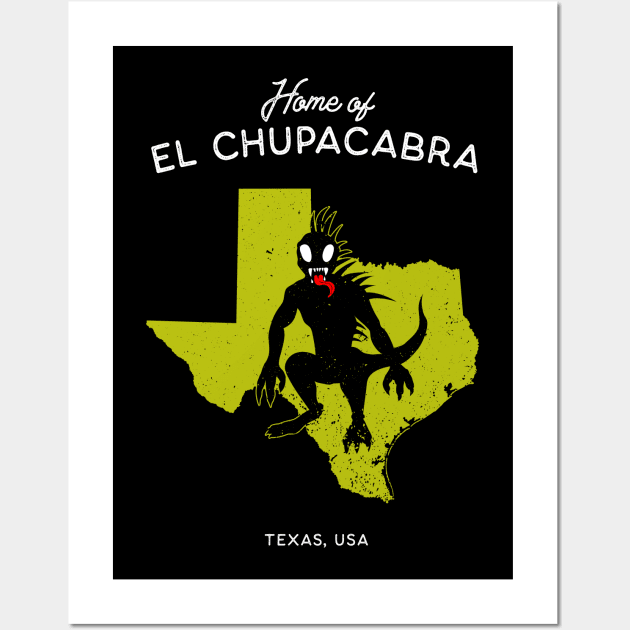The poster features a striking design with a thick white border framing a black background. At the top, in white lettering, are the words "Home of El Chupacabra," with "Home of" in a script font and "El Chupacabra" in bold capital letters, slightly arched from left to right. Centered on the poster is a vivid yellow outline of the state of Texas, rendered in a slightly distressed style that allows hints of black to show through. Superimposed over Texas is a menacing depiction of the Chupacabra. This creature, appearing almost like a swamp monster or demon, is crouched with its three-toed lizard-like feet and front limbs that resemble arms jutting from its shoulders. 

The Chupacabra has an elongated alien-like head with long, perpendicular white oval eyes. Sharp yellow teeth gleam from its gaping mouth, from which a vivid red lizard-like tongue protrudes. Along its back and head are pronounced, dinosaur-like spikes. The creature’s silhouette is detailed in black, with elements overlapping the Texas outline accented in bright green, adding to its eerie presence. Completing the image, "Texas, USA" is written in smaller white capital letters at the bottom of the poster. The backdrop behind the poster is a very pale gray, adding to the stark and intense visual impact.